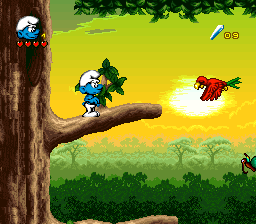In this image, we are looking at a small, detailed still from a video game featuring the Smurfs. Dominating the left-hand side of the frame is a large, verdant tree with a prominent branch extending outward. Perched on this branch is a blue Smurf, easily identifiable by his white hat and boots. In the bottom-left corner of the frame, a small portrait of a Smurf's face is visible, accompanied by four tiny red hearts below it, indicating the remaining lives in the game.

Front and center, approaching the Smurf, is a vibrant red bird in mid-flight. The top right-hand corner contains a mysterious white streak, next to which is the number 9, possibly indicating a game score or level.

The background is a picturesque forest scene featuring a glowing sun and lush green trees, adding a sense of depth and natural beauty to the setting. A black bird appears to be flying through this richly animated forest, adding to the dynamic nature of the scene. In the bottom right-hand corner, part of another tree branch is visible, sneaking into the frame and contributing to the overall forested atmosphere.